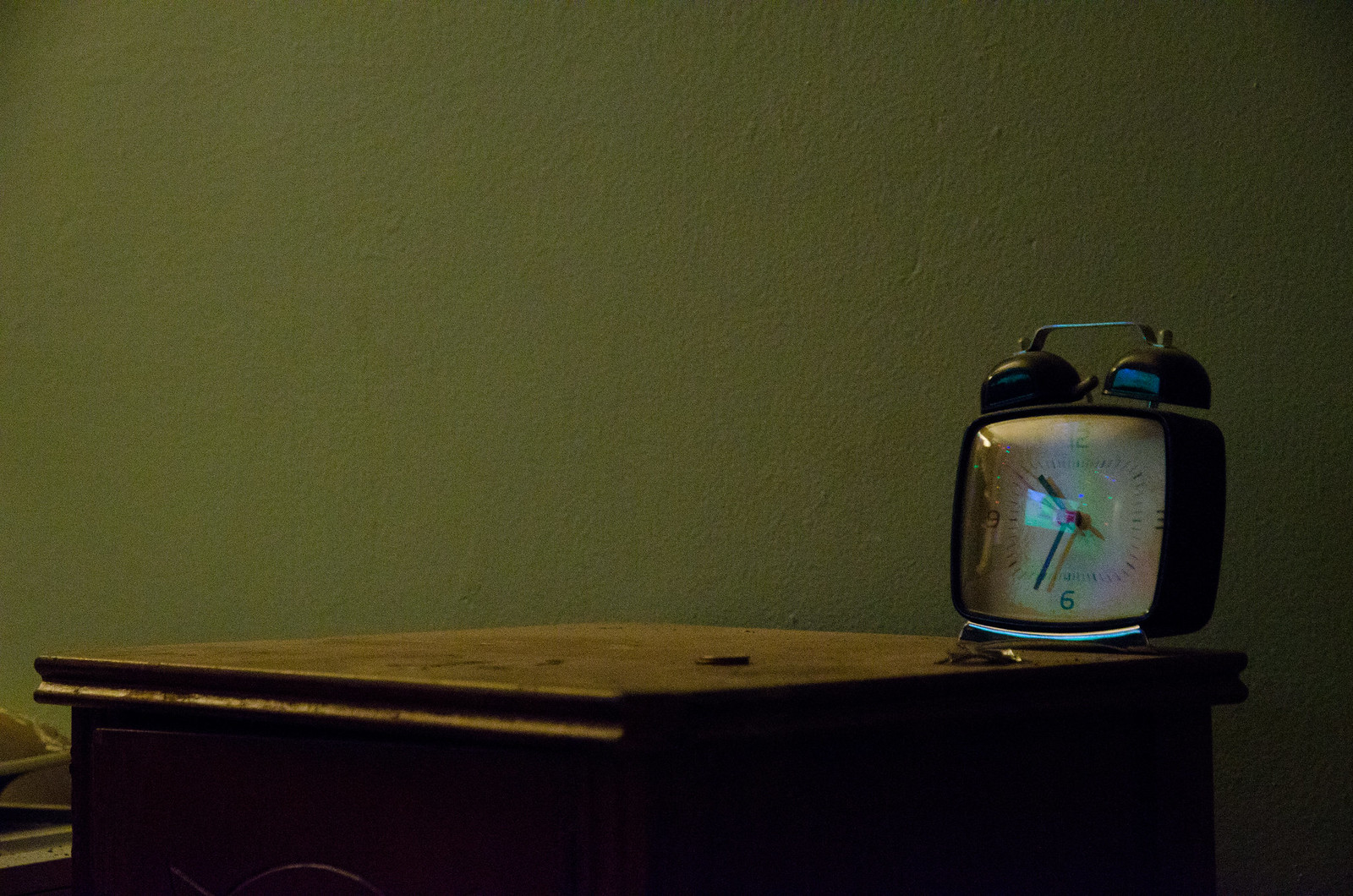The dimly lit indoor photo captures a serene bedroom setting featuring white walls that form a neutral backdrop. In the foreground, a rustic wooden nightstand with a smooth, flat surface stands prominently. At the corner of the nightstand rests a vintage alarm clock. The clock is square-shaped with a distinctive design—two silver bells perched on top, connected by a slender rod. Encased in glass, the clock face is white, featuring bold black numbers at 12, 3, 6, and 9 positions, with simple lines marking the other hours. The hour and minute hands are black, while the seconds hand is a striking red, adding a subtle touch of color to the otherwise monochromatic scheme.